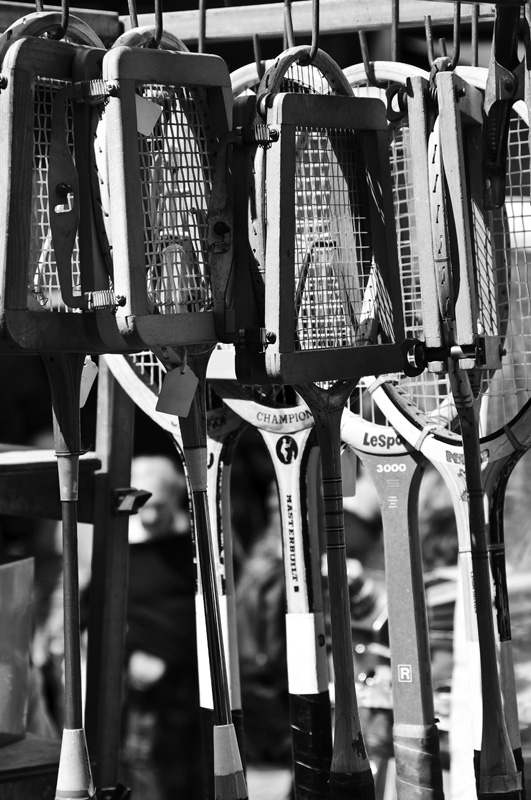This vertically shot black and white photograph showcases a row of old-fashioned wooden tennis rackets, meticulously hung on black metal hooks. The rackets, numbering at least eight, are displayed in wooden racket presses designed to prevent warping, adding a vintage charm to the composition. The rackets' handles, some featuring striped patterns and others solid wood, suggest signs of use. Prominent among the visible brand names are "Champion" and "Le Sportif," while some inscriptions are partially obscured. The artful lighting of the photograph casts dramatic shadows, enhancing the texture and details of the rackets. In the blurred background, faint outlines of people are discernible, suggesting a bustling environment, possibly a sports shop or storage facility. The square-shaped elements on some rackets further emphasize the retro appeal of this evocative image.